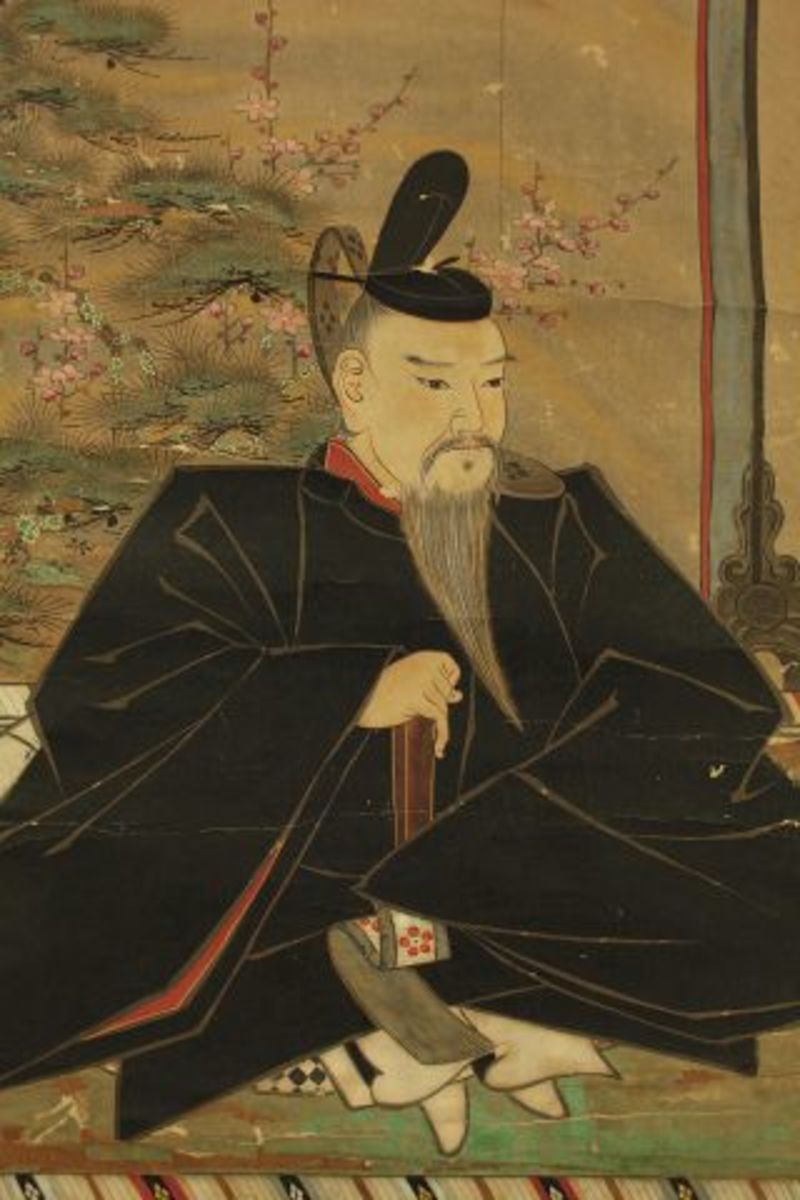The image is a detailed drawing of an ancient Chinese man, presented in a rectangular format resembling a renowned piece of traditional artwork, possibly painted on fabric, as indicated by a fold at the top of the picture. The man, depicted with fair skin and an even tone, exudes a stern demeanor. He has a thin gray mustache and a long beard that reaches below his chest. His downcast eyes contribute to his contemplative expression. He wears a small circular black hat with a long black extension resembling an open flap or stylized ponytail at the back. His attire consists of a large, flowing black robe with a red collar and underlay, similar to a graduation gown, adorned with extraordinarily long and wide sleeves.

The man sits cross-legged on a greenish-brown mat, with one hand gripping a wooden belt featuring a green bottom part and a red flower pattern in the white area on the green part. Behind him, the backdrop showcases an ornate scene depicting green trees and pink cherry blossoms, with mountains in shades of gray-green, hinting at a tranquil natural setting. This painting captures both the intricate details of his traditional attire and the serene, yet noble ambiance of the background.